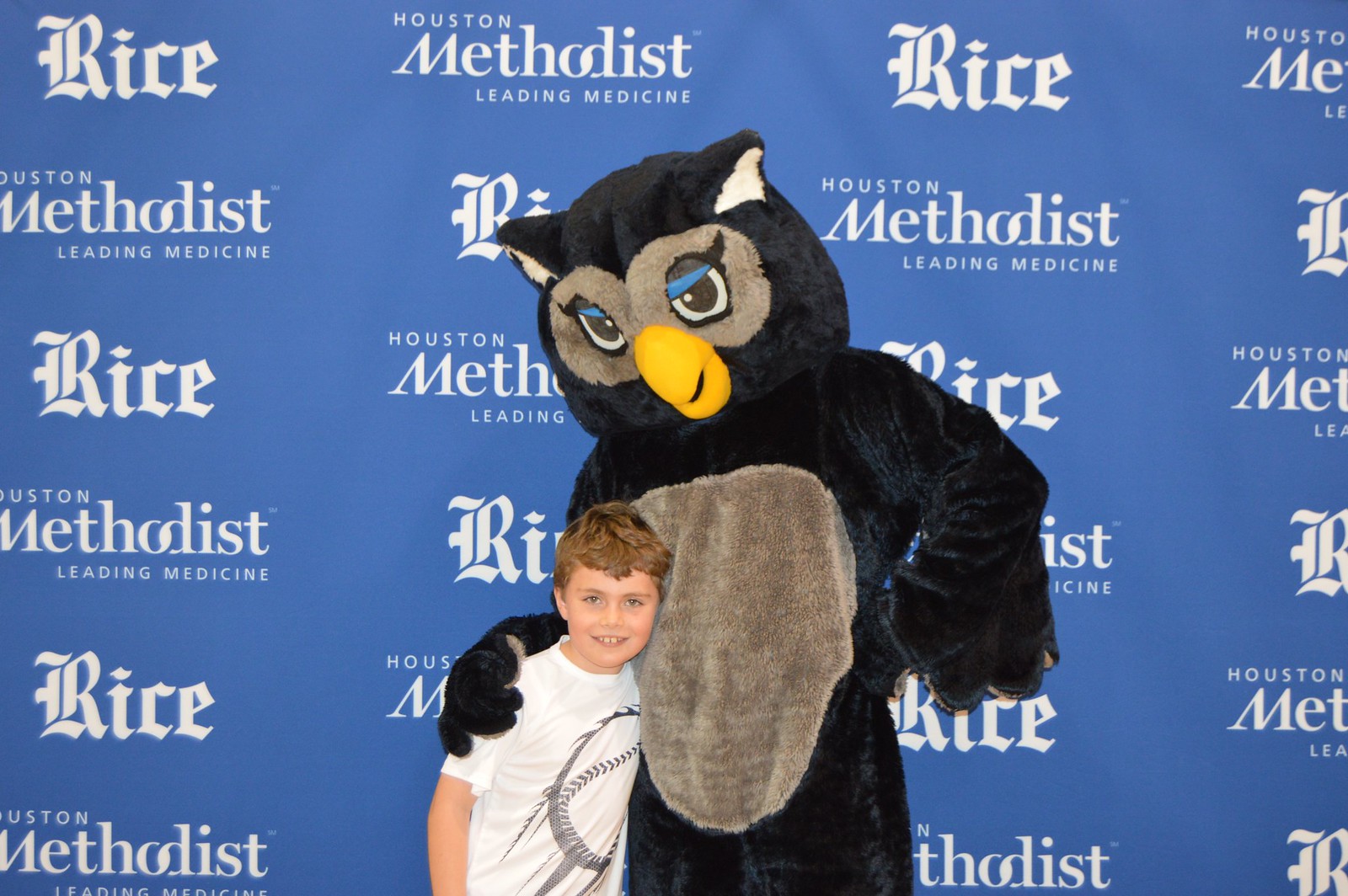In this image, a young Caucasian boy with short brown hair, wearing a white short-sleeve t-shirt adorned with a baseball graphic, is smiling joyfully at the camera. He is being gently held by a mascot designed to resemble an owl. The owl costume predominantly features black fur, a light gray stomach area, a yellow beak, and brown patches around its eyes, providing it with a distinct avian appearance. This heartwarming interaction takes place against a blue background adorned with repeating logos of "Rice" and "Houston Methodist Leading Medicine," emphasizing a celebratory or promotional setting tied to these institutions.